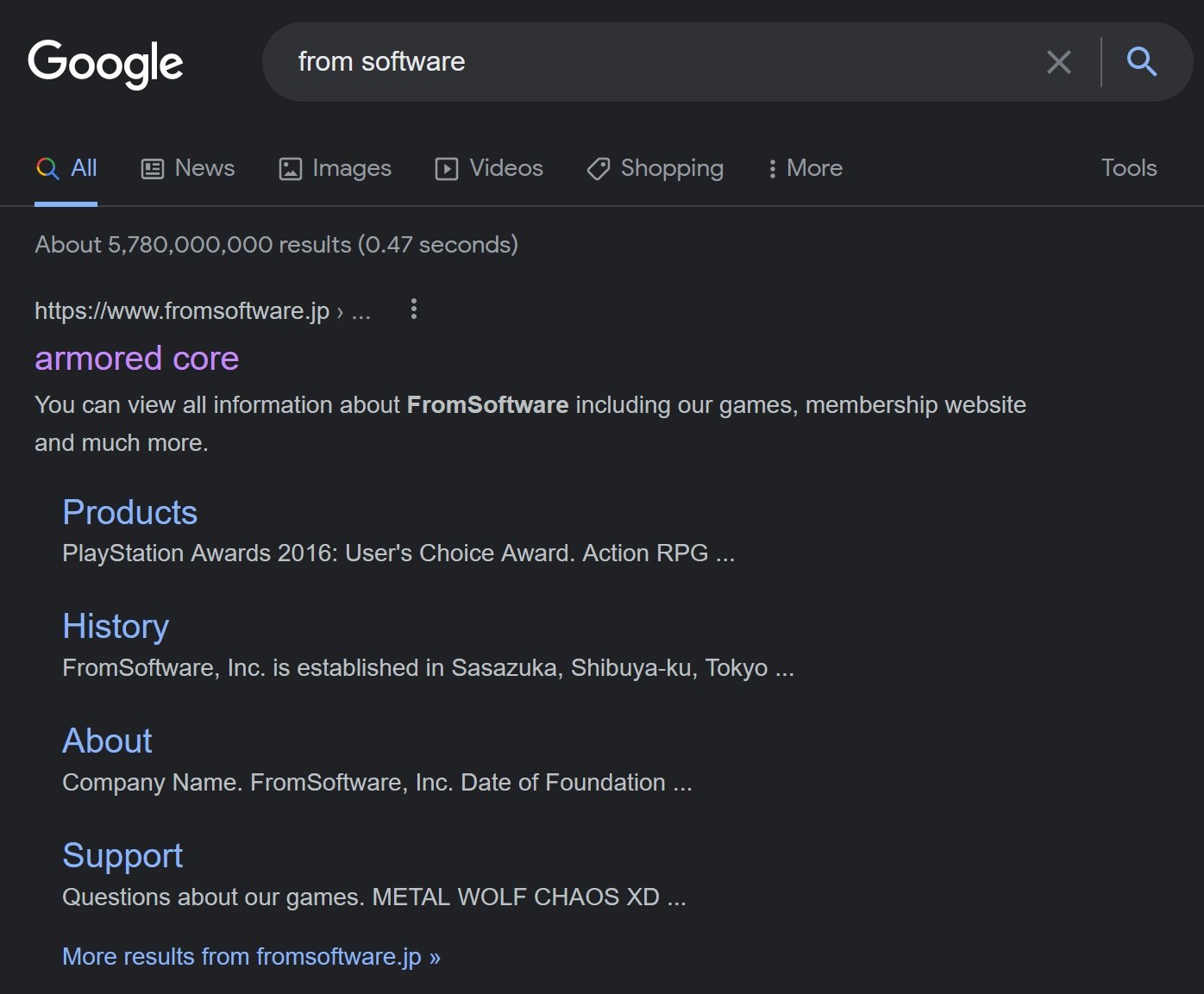The image displays a Google search interface set against a black background, likely indicating the use of a dark mode setting. The scene could be on either a laptop or a phone, though no specific indicators confirm the device type. The prominent white Google logo is positioned in the top left corner, adjacent to an elongated search bar that extends from the top center to the top right of the screen. Inside the search bar, the phrase "from software" is typed in lowercase white text.

Below the search bar are category options arranged from left to right: All, News, Images, Videos, Shopping, and More. The search results are visible, with the first result focusing on "Armored Core," followed by additional tabs labeled Products, History, About, and Support. Each of these tabs features blue icons, except for "Armored Core," which is highlighted in purple, indicating that it has been previously accessed by the user.